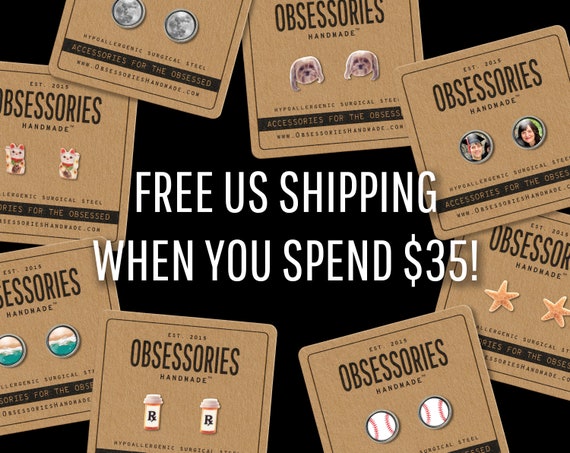The advertisement for Obsessories, a company established in 2015, showcases various charm-like earrings made from hypoallergenic surgical steel, displayed on simple brown backing cards with the company’s printed information. The ad, set against a black background, prominently offers free U.S. shipping for purchases over $35. Featured earring designs include a graduate and a mother, starfish, baseballs with red stitching, pharmacy pill containers (RX), a sunset ocean scene with turquoise water and clouds, an Asian cat with a moving arm, the moon, puppies, and pink and white kittens. The assortment highlights the diversity and whimsical nature of the designs offered by Obsessories.